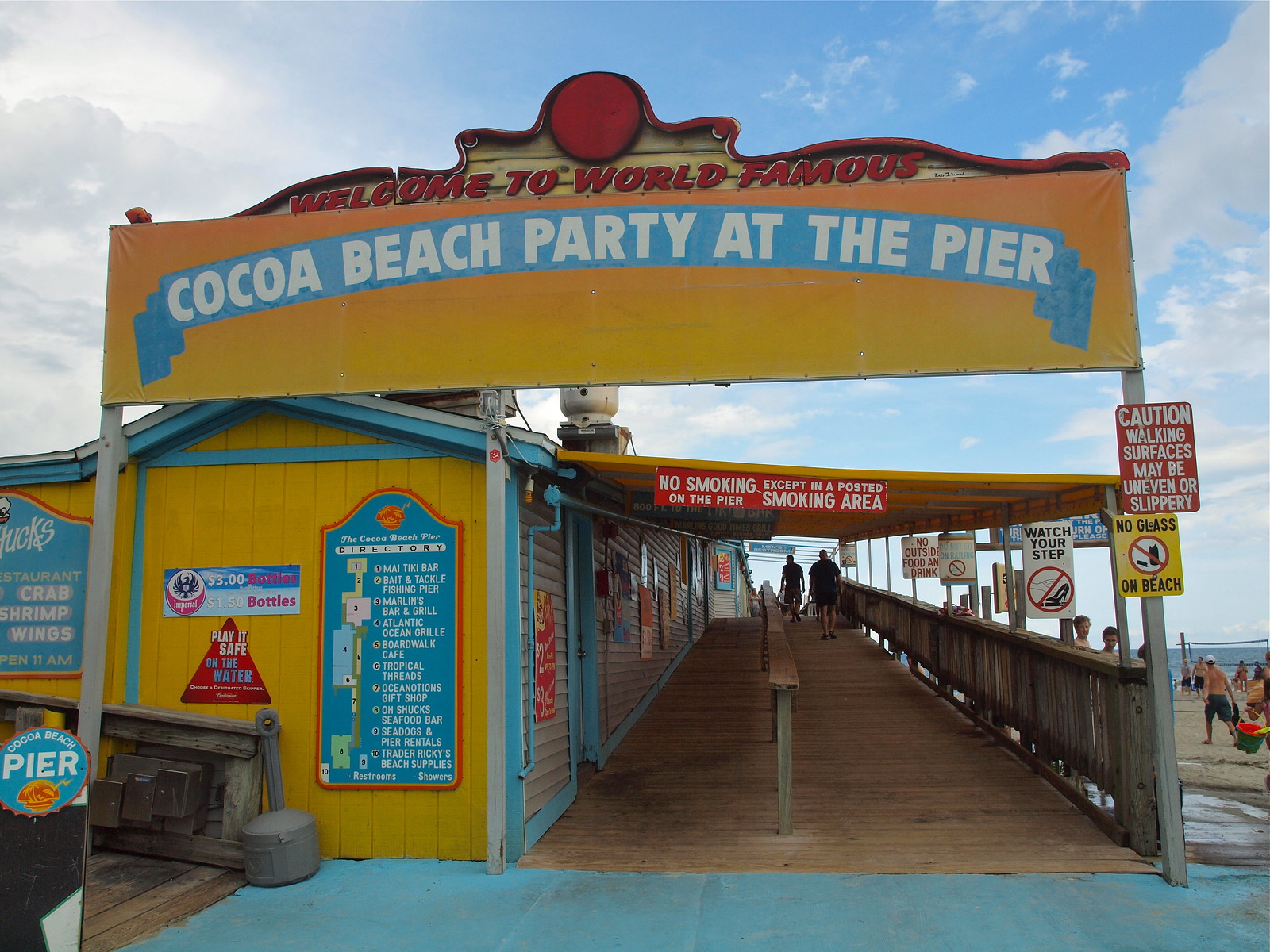The image captures a bustling scene at the entrance to the Cocoa Beach Pier. A prominent wooden ramp leads up to a yellow-sided building with blue trim, which houses various shops and eateries. Above the ramp, a large wooden sign reads, "Welcome to the World Famous Cocoa Beach Party at the Pier," with a fancy blue scroll and white lettering set against a yellow background. Hanging from the roof above the ramp are numerous signs stating various regulations such as "No smoking on the pier except in a posted smoking area," "Caution: walking surfaces may be uneven or slippery," "No glass on beach," "Watch your step," "Do not sit on the railing," and "No outside food or drink."

Beneath these signs, a directory lists several attractions including My Tiki Bar, Bait and Tackle Fishing Pier, Marlins Bar and Grill, Atlantic Ocean Grill, Boardwalk Cafe, Tropical Threads, Ocean Notions Gift Shop, O'Shuck's Seafood Bar, Sea Dogs and Pier Rentals, and Trader Ricky's Beach Supplies. The pier area is lively, with people in swimsuits walking up the ramp, some carrying buckets and shovels for building sandcastles. A volleyball net is visible in the background, and the sky is partly cloudy with a hint of blue, adding to the vibrant, tourist-friendly atmosphere of the scene.